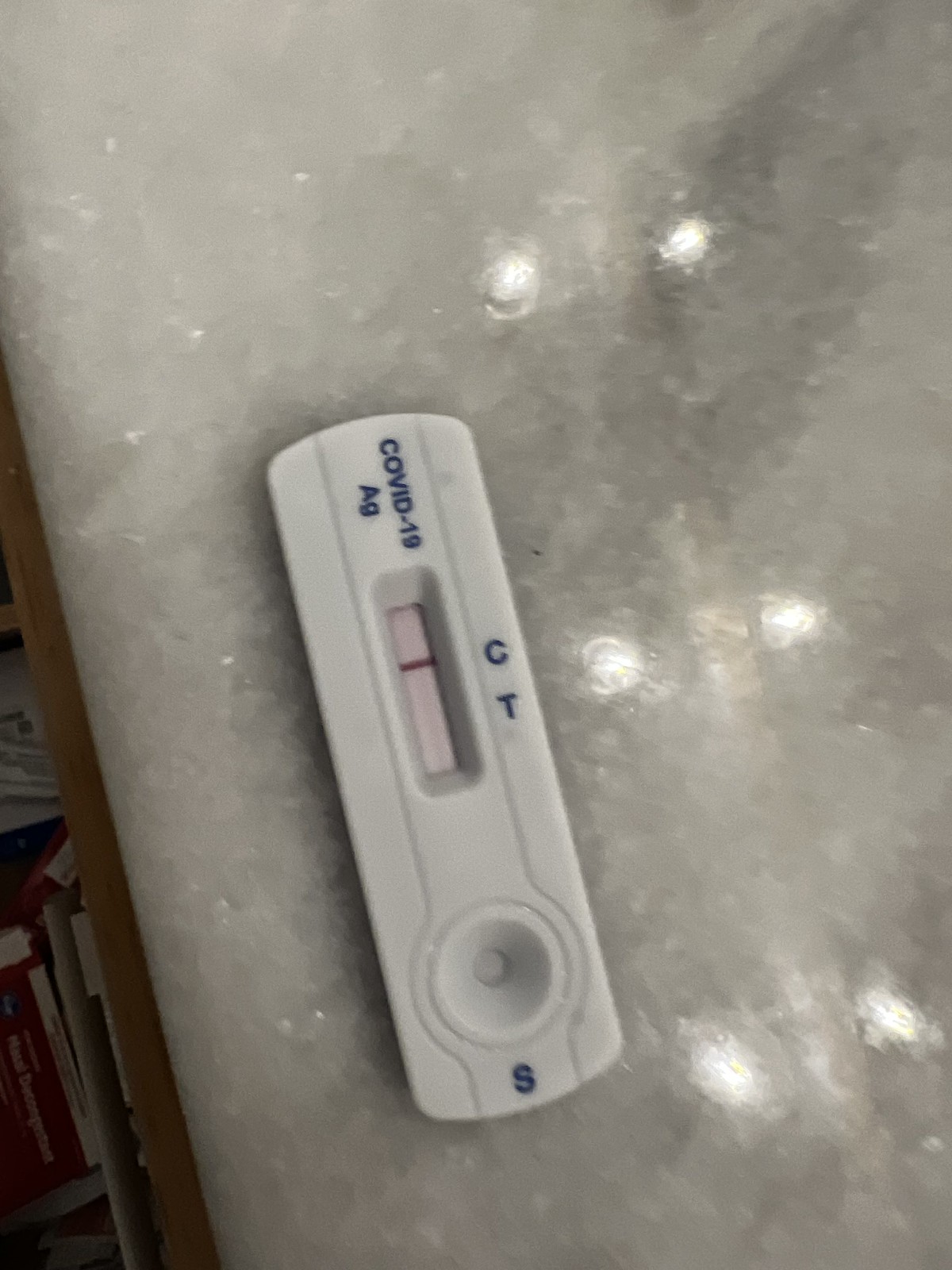A detailed photograph captures a view from above of a reflective white surface, likely made of marble or quartz, showcasing its smooth, glossy finish with subtle gray veining and a scattering of lighter specks that lend it a sparkling appearance. The surface reflects light from six distinct sources above, enhancing its pristine look. In the lower region of the image, a clutter of items is visible, including a box of files, assorted paperwork, red boxes, and white folders, hinting at a disorganized area, perhaps atop a shelf. Central to the composition is a small, plastic COVID-19 antigen test, predominantly white with blue lettering that reads "COVID-19 AG." The test features a rectangular window displaying a single red control line, indicating a negative result as the test line remains blank. Below the window, an "S" marks the spot where the sample liquid is applied, completing the practical yet detailed scene.